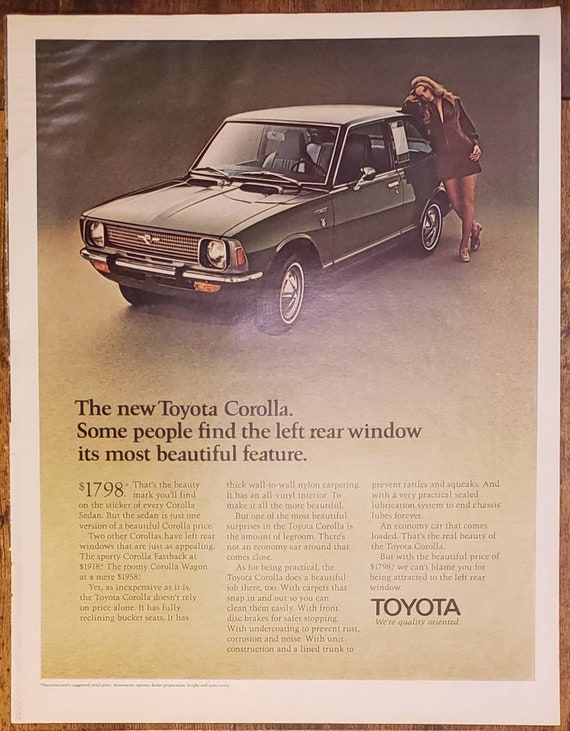This advertisement is a vintage Toyota ad, likely from the 1970s, featuring a striking visual and detailed text that harks back to the era's print magazine style. It is a vertically aligned rectangular sheet of paper with a distinct white border set against a wooden surface. The focal point of the ad is an image at the top of a dark-colored, possibly green or dark grey, Toyota Corolla, which resembles a hatchback.

Leaning on the car with a casual elegance is a beautiful blonde-haired model wearing a brown dress, which features a zipper down the center. She is posed with her elbow resting on the hood and her head on her arm, her legs crossed, and one hand on her hip. The dress is short, and she is wearing heels that may be green or grey in color.

Directly underneath the image of the car and model, the text states in bold lettering, "The new Toyota Corolla. Some people find the left rear window its most beautiful feature," referring to the appealing design of the car. Below this headline, three paragraphs of smaller text provide additional information about the vehicle. The ad concludes with a large, bold "TOYOTA" at the lower right corner, accompanied by the tagline, "We're quality-oriented," emphasizing the brand's commitment to excellence.

Overall, the advertisement effectively combines visual allure with informative content, capturing the essence of vintage automotive advertising.